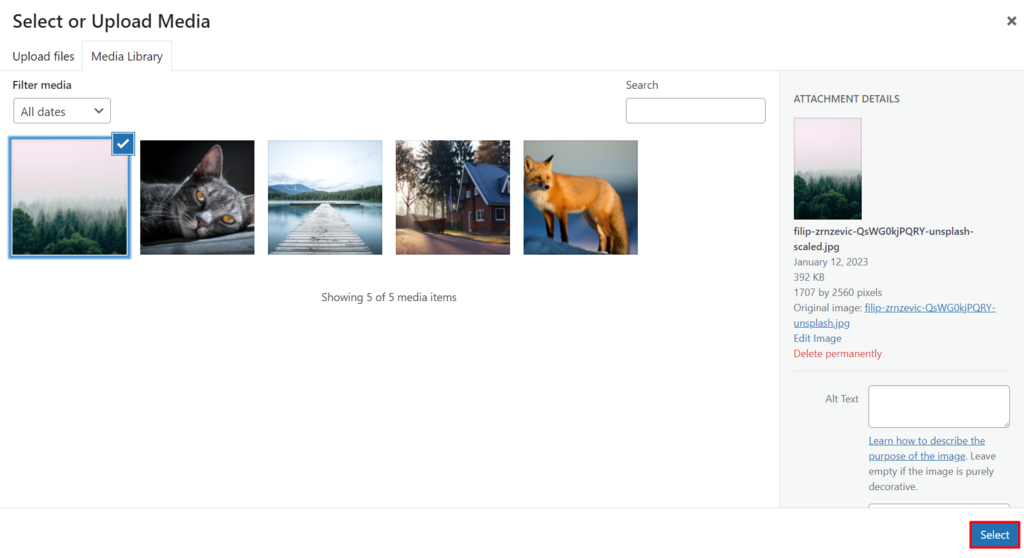This image is a cropped screenshot of an attachment page interface within a media library. Dominating the top-left corner in bold black text is the prompt "Select or upload media." Directly below are two navigational tabs labeled "Upload Files" and "Media Library." Further down, in smaller black font, is the text "Filter media" accompanied by a dropdown box currently set to "All dates."

The user sees five image thumbnails arranged in a row, with the first thumbnail—depicting a misty mountain scene—selected. In the top-right corner of the interface, there is a search bar allowing for quick navigation through media items. The bottom end of the thumbnail section indicates, "Showing 5 of 5 media items," confirming the total number displayed.

On the right side of the screen, a gray panel titled "Attachment Details" provides comprehensive information about the selected image. Central to this panel is the thumbnail itself, surrounded by detailed metadata, including the file name, location, date, and size, as well as the original image link. Below these details, two actionable options are available: "Edit Image" in blue and "Delete Permanently," highlighted in red. Additionally, there is a text field labeled "Alt Text," accompanied by a sizeable input box for adding alternative text.

At the bottom-right corner of the screen, a small blue button labeled "Select" has been visually emphasized with a red box around it, highlighting its importance.